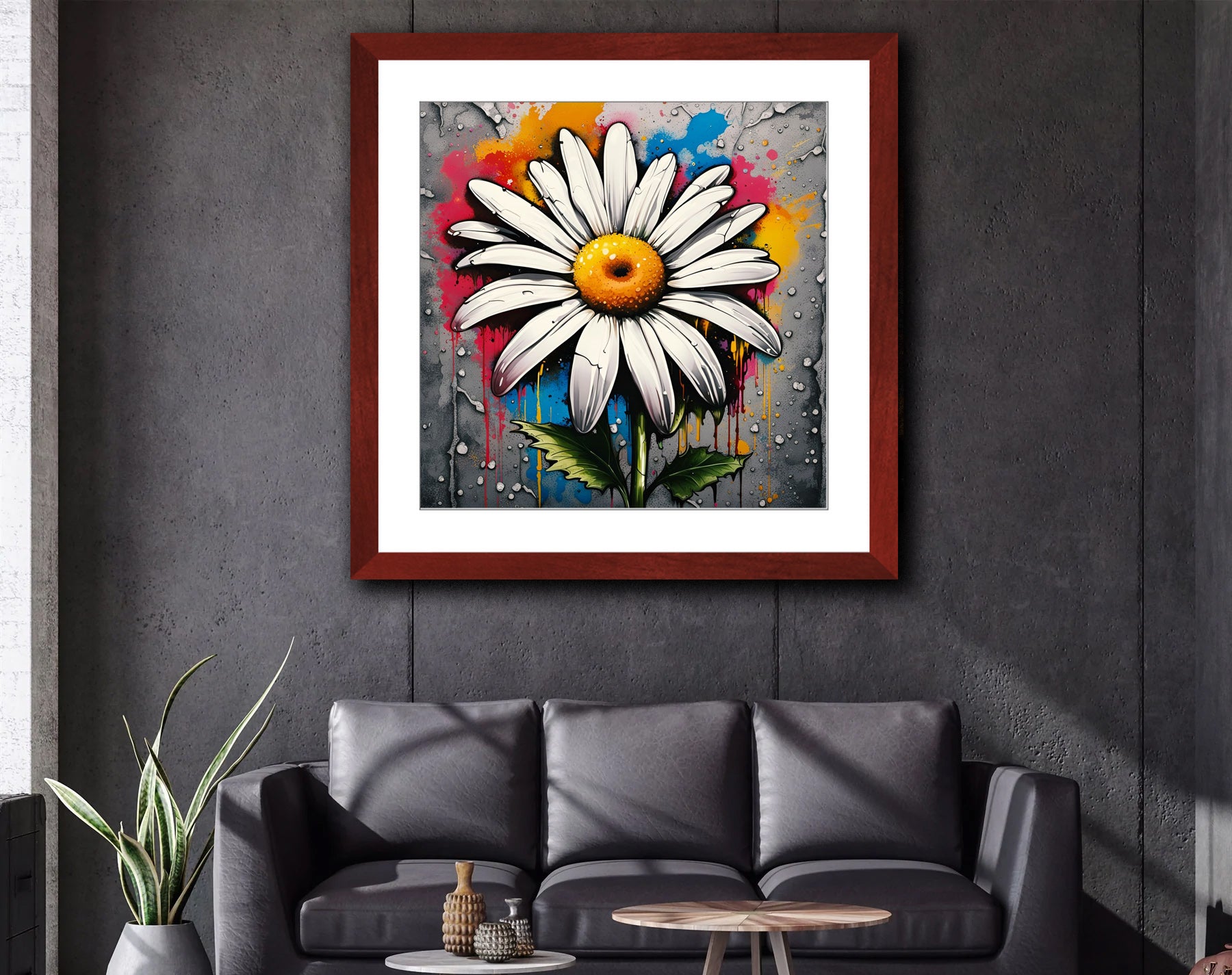The photograph showcases a modern living room centered around a striking wall artwork. The painting, framed in a reddish wood (possibly redwood or mahogany) frame with a white border, depicts a cartoon-styled white daisy with a light green stem and a yellow center, all set against a vivid tie-dye backdrop featuring hues of red, pink, blue, and orange. This colorful design contrasts with the gray background, giving the impression of dripping paint and water droplets. The artwork hangs on a gray concrete wall above a black leather three-seater couch, which has three cushions and three pillows.

In front of the couch, there are two small round tables: a larger wooden table and a smaller white table with a marble top. The white table holds three decorative vases. To the left of the couch is a gray circular planter with long green leaves, while to the right, sunrays filter through a nearby window, subtly illuminating the scene. The meticulously arranged space combines elegance and a touch of playfulness, creating a visually engaging setting.